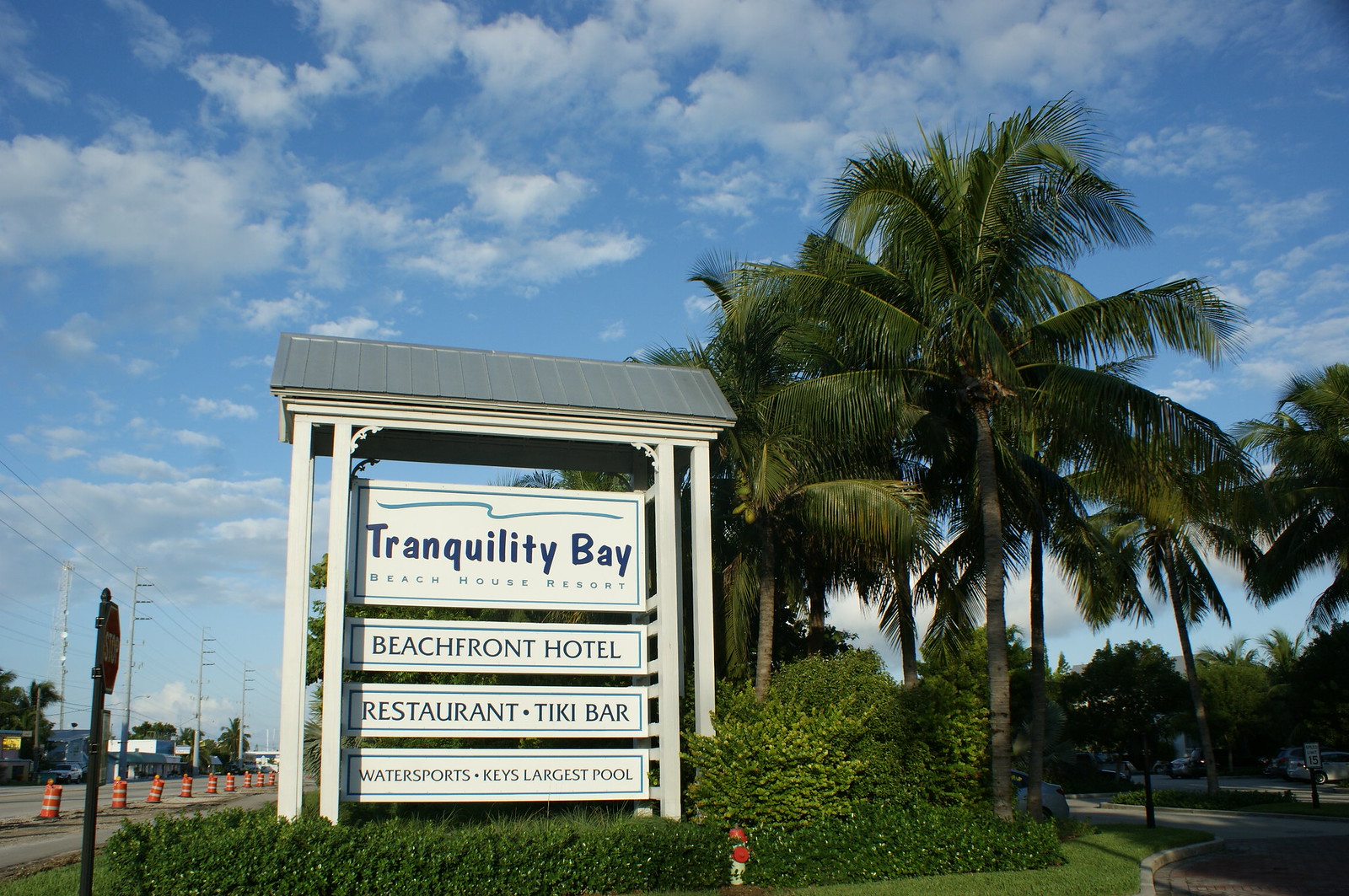The image captures a vibrant outdoor scene showcasing a bright and colorful street sign. The sign, situated on a green, landscaped island, features a sturdy, gray housing roof with supporting beams. Below the roof, there are four rectangular, white signboards arranged vertically. The top signboard prominently displays the name "Tranquility Bay Beach House Resort" in bold blue letters. The subsequent boards read "Beachfront Hotel," "Restaurant Tiki Bar," and "Watersports - Keys Largest Pool," albeit the text on some boards is quite small and difficult to read. 

Surrounding the sign, lush green grass and bushes accentuate the tropical ambiance, while several tall palm trees line both the green island and the adjacent sidewalk. To the left of the sign, a paved road bordered with orange construction cones is visible. On the right, a cobblestone pathway or driveway adds to the picturesque setting. The backdrop is dominated by a clear blue sky, adorned with thin, calm white clouds, contributing to the serene and inviting atmosphere of this beachside locale, presumably the Florida Keys. In the distant background, a speed limit sign can also be glimpsed, adding to the overall detailing of the streetscape.